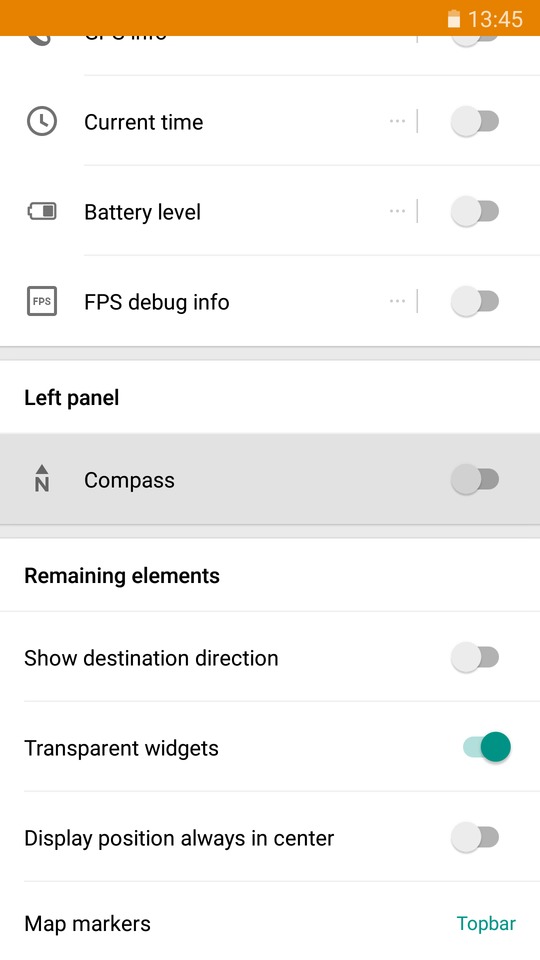Screenshot from a mobile device displaying a settings menu in a white background theme. At the top left corner of the screen, there is a time display and a power indicator showing the remaining battery life, both situated on an orange strip. Below this strip is an account section from a website or app interface, featuring a list of toggle options that allow the user to turn various settings on or off.

The settings options are as follows:

1. Current Time (with a clock icon next to it)
2. Battery Level (with a battery icon next to it)
3. FPS Debug Info (with a square box around the letters "FPS")
4. Left Panel
5. Compass (highlighted in gray)
6. Remaining Elements
7. Show Destination Direction
8. Transparent Widgets
9. Display Position
10. Always in Center
11. Map Markers

Each option is listed in black text with an on/off toggle switch on the right side. Currently, all options are toggled off except for "Transparent Widgets," which is highlighted with a teal blue switch indicating it is turned on. Additionally, "Map Markers" has a unique hyperlink labeled "Top Bar" in blue text, instead of a toggle switch. 

This detailed menu likely allows the user to customize various visual and functional elements of their mobile app or website interface.